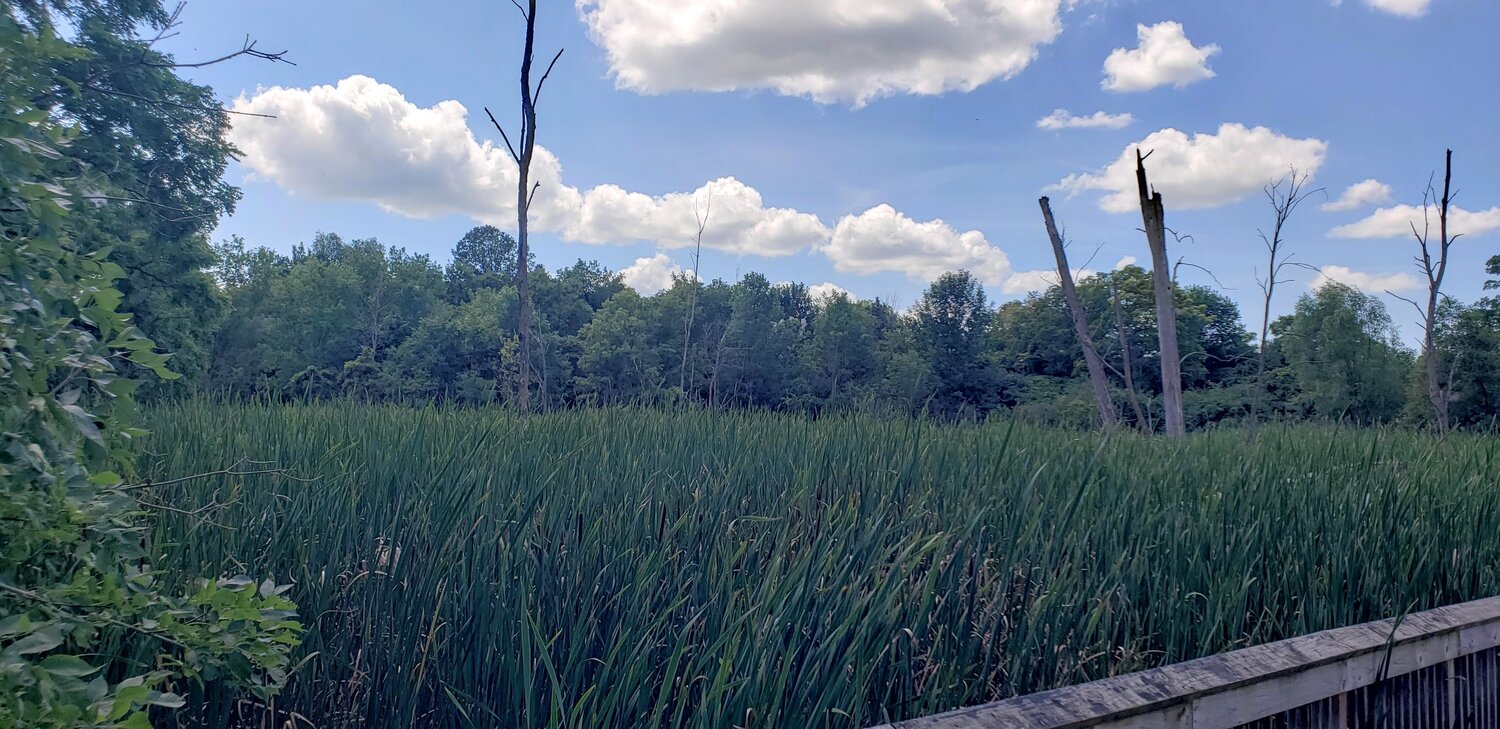This serene outdoor nature photograph was captured from a wooden walkway traversing a swampy area, evidenced by the wooden railing in the bottom right corner. The foreground is dominated by tall, green grasses and reeds characteristic of wetlands, standing taller than the railing itself. Among the lush greenery, several tree trunks and branches appear lifeless, likely having succumbed to overwatering after the area transformed into a wetland. These bare, skeletal trees contrast starkly with the vibrant, full-canopied trees visible to the left and in the background, creating a fascinating juxtaposition of life and decay. The sky above features a mix of high, fluffy white clouds interspersed with patches of clear blue sky, adding a tranquil, airy quality to the scene. The setting is utterly devoid of animals or people, inviting a sense of calm and solitude.